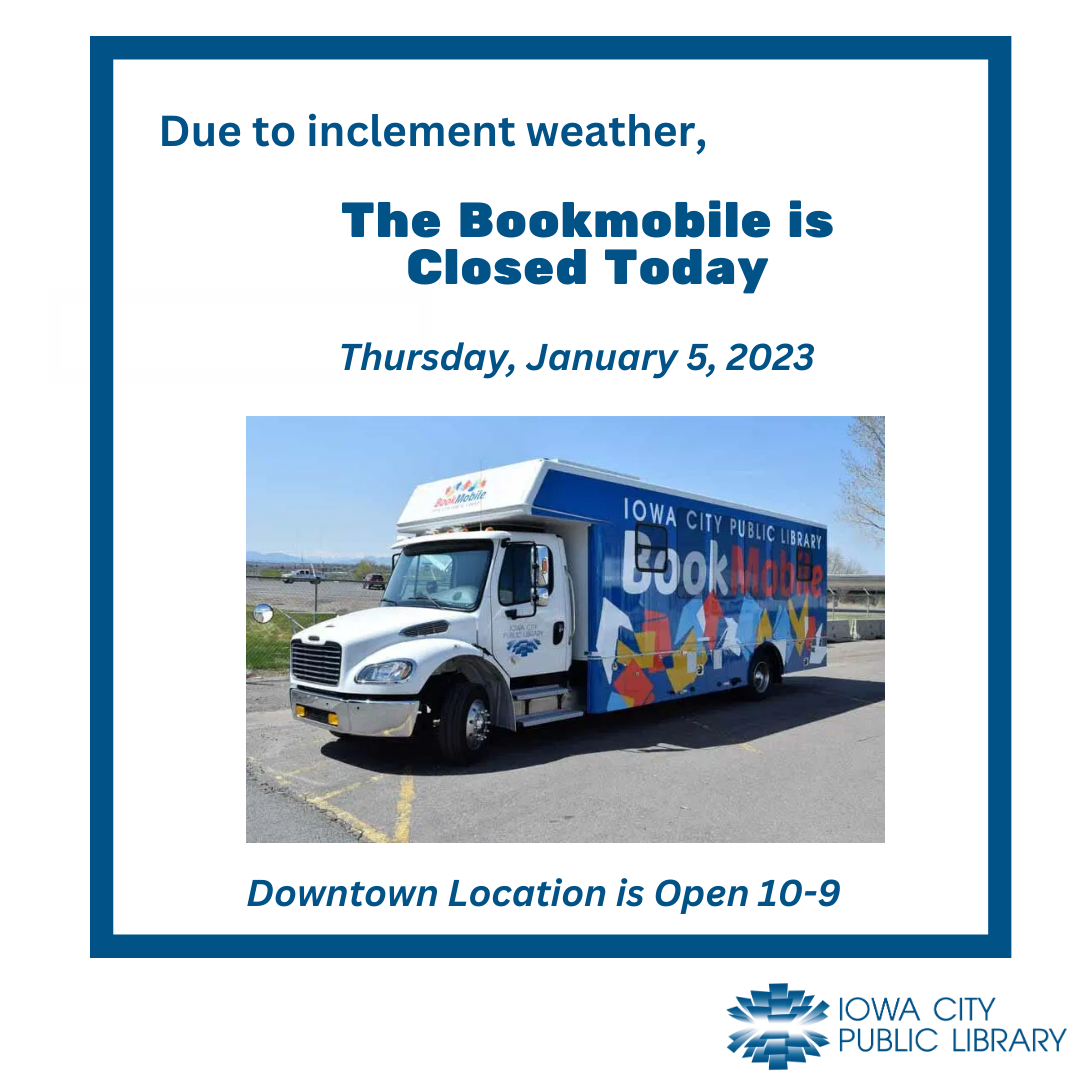This image features an announcement from the Iowa City Public Library. Set against a white background, the announcement includes both text and a photograph, all framed by a blue border that extends around most of the image. Outside the blue border, in the lower right corner, is the Iowa City Public Library logo. 

The text inside the blue-bordered box announces in blue font: "Due to inclement weather, the Bookmobile is closed today, Thursday, January 5th, 2023." Below this announcement, a photograph of the Bookmobile is displayed. The Bookmobile is a large truck with a white cab. The rear section of the truck is blue, adorned with white and red decorations, and bears the words "Bookmobile" in bold white text at the top, along with "Iowa City Public Library." 

Underneath the photograph, small blue text informs readers that the "Downtown location is open 10 to 9." This detailed notice is intended to inform the residents of Iowa City about the closure of the Bookmobile due to weather conditions while also providing information that the downtown library location remains open.